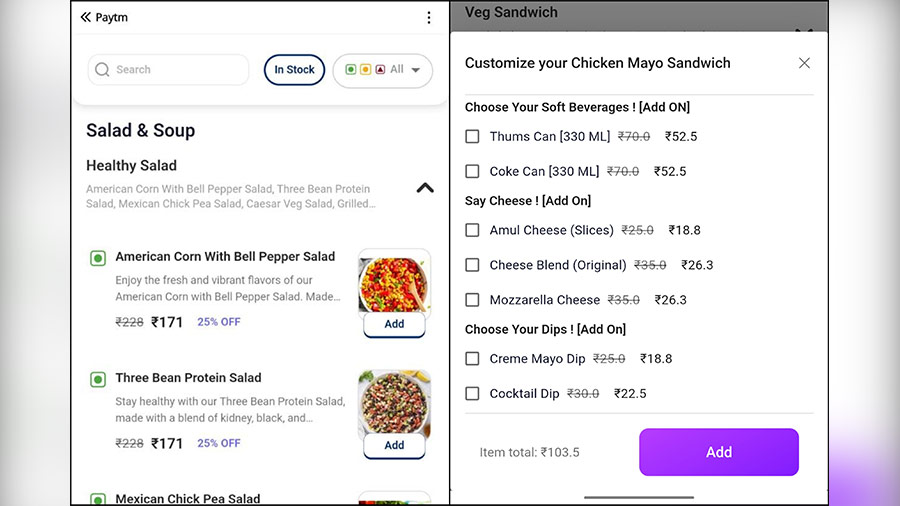This image is a screenshot from an online ordering application, PayTM. In the top left corner, the PayTM logo is displayed along with two left-pointing arrows indicating navigation options. Below the navigation bar, there is a searchable area with options to filter items in stock and sort by various criteria.

The primary section of the screenshot focuses on a submenu titled "Salad and Soup," highlighting three salads under the "Healthy Salad" category. The visible salads include:
1. **American Corn with Bell Pepper Salad** – represented with an accompanying image.
2. **Three Bean Protein Salad** – also shown with an image.
3. **Mexican Chickpea Salad** – the image is partially cut off in the screenshot.

Alongside this, there is a sidebar listing "Veg Sandwich," where the user is prompted to customize their order for a "Chicken Mayo Sandwich." Additional options are available for an extra charge, including a variety of soft beverages. Below these selections, the itemized total bill is displayed, amounting to 103.5.

Specific customization options for the Chicken Mayo Sandwich include:
- Choice of drinks
- Cheese options
- Mayo variations
- Cocktail dip

This detailed overview provides a comprehensive picture of the online ordering interface and options available to the customer.